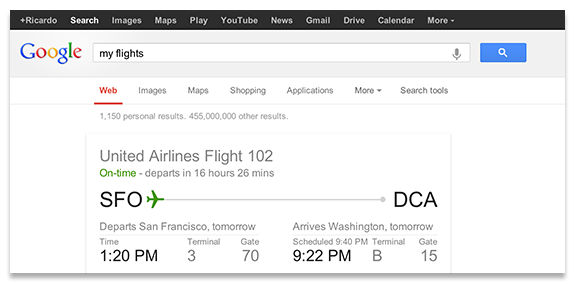This image is a cropped and minimized screenshot of a Google desktop page. The visible portion reveals a slight grey background beneath the bottom, left, and right edges of the main content window, giving the impression that the box is raised due to subtle shading. The top of the screenshot features a grey header with the "Google" logo situated on the left side. To the right of the logo, there is a search bar containing the query "my flights."

Below the header, the main body of the Google webpage is predominantly white. The page reveals that the search has yielded two sets of results: 1,150 personal results and 455 million other results, both displayed in small grey letters beneath the search bar. The content prominently displays a United Airlines flight 102, indicating that the flight is on time and scheduled to depart in 16 hours and 26 minutes. Additional flight information is also shown, likely specific details about the itinerary.

The image suggests that the user has typed "my flights" into Google, which has returned personal information related to their accounts. The presence of personal flight details indicates the individual's heavy usage of Google services, including possibly multiple Google accounts contributing to the personal information displayed.